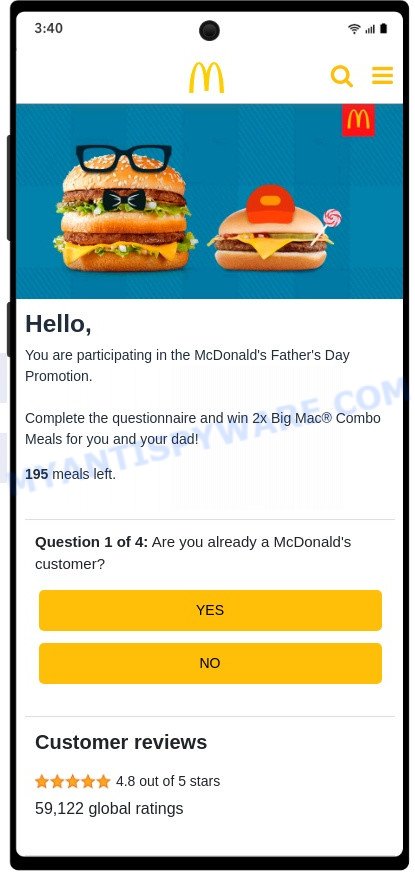The image features a white background and a prominent yellow "M" for McDonald's at the top. The time displayed is 3:40. Below the logo is a yellow search bar and a yellow hamburger icon. The image incorporates two cartoon burgers: one resembling a Big Mac adorned with a bowtie and glasses, and the other, a smaller cheeseburger, wearing a red cap and holding a red and white lollipop.

Text in the image announces participation in a McDonald's Father's Day promotion, offering a chance to win double Big Mac combo meals (2x) for you and your dad upon completing a questionnaire. It notes the availability of 195 meals left. Question 1 of 4 asks, "Are you already a McDonald's customer?" and offers two yellow rectangles as response options—one saying "Yes" in black, and the other saying "No" in black. Customer reviews indicate a high satisfaction with 4.8 out of 5 stars from 59,122 global ratings.